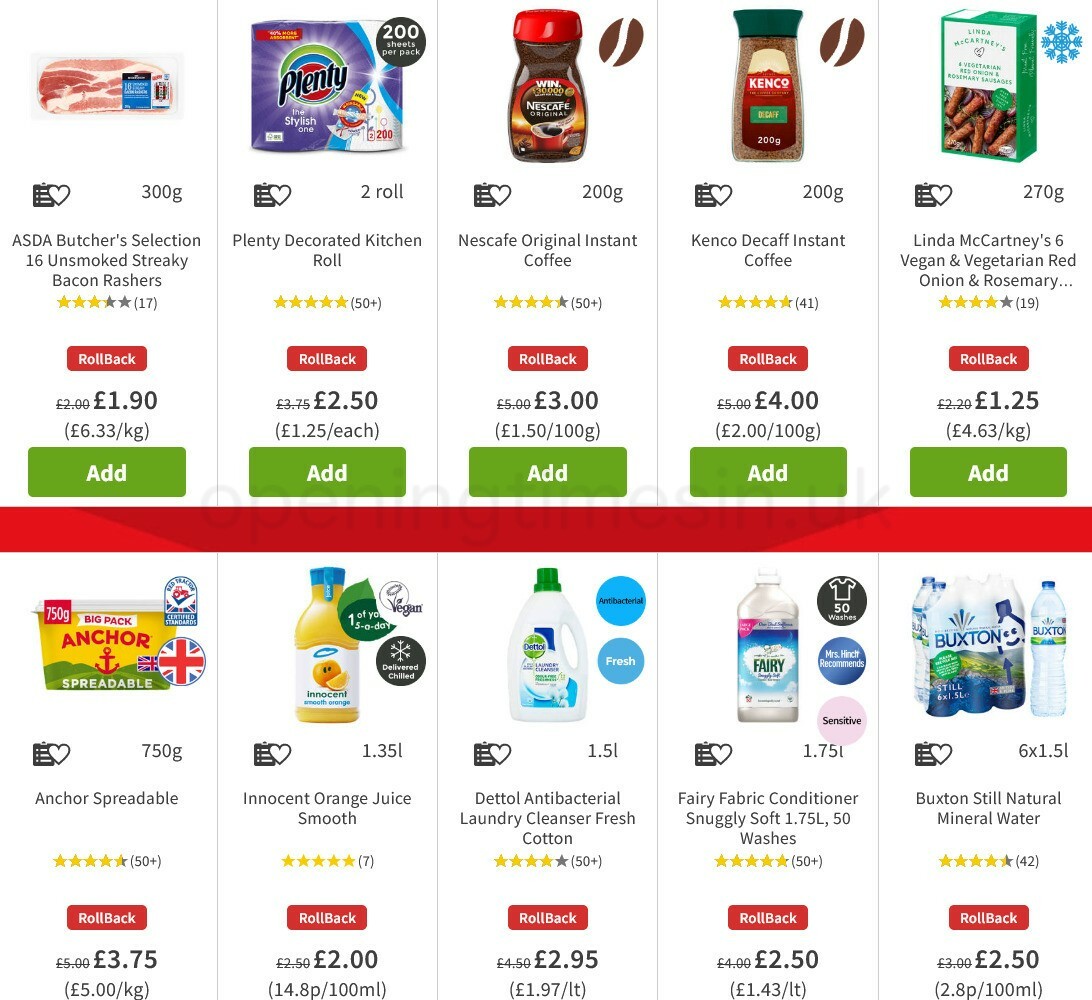This web page appears to be from a grocery store, possibly Instacart or ASDA. It showcases 10 different food and household items available for purchase, all with rollback prices, giving a sense of a discount or special offer. Below is a detailed description of each item:

1. **ASDA Butcher's Selection Unsmoked Streaky Bacon Rashers**: 
   - Price: £1.90
   - Quantity: 16 rashers
   - Weight: 300g
   - Rating: 3 stars based on 17 reviews
   - Note: Rollback price

2. **Plenty Decorated Kitchen Roll**:
   - Price: £2.50
   - Type: Paper towels
   - Note: Rollback price

3. **Nescafe Coffee**:
   - Description and details are not provided

4. **Kenco Decaf Coffee**:
   - Description and details are not provided

5. **Linda McCartney's Vegan and Vegetarian Red Onion and Rosemary Crackers**:
   - Quantity: 6 crackers
   - Description details not provided
   - Note: Rollback price

6. **Anchor Spreadable**:
   - Description and details are not provided
   - Note: Rollback price

7. **Innocent Orange Juice Smooth**:
   - Description and details are not provided
   - Note: Rollback price

8. **Dettol Antibacterial Laundry Cleanser, Fresh Cotton**:
   - Description and details are not provided
   - Note: Rollback price

9. **Fairy Fabric Conditioner, Snuggly Soft**:
   - Description and details are not provided
   - Note: Rollback price

10. **Buxton's Still Natural Mineral Water**:
    - Description and details are not provided
    - Note: Rollback price

Each item can be easily added to the shopping cart, making it convenient for users to shop for groceries and household essentials at discounted prices.